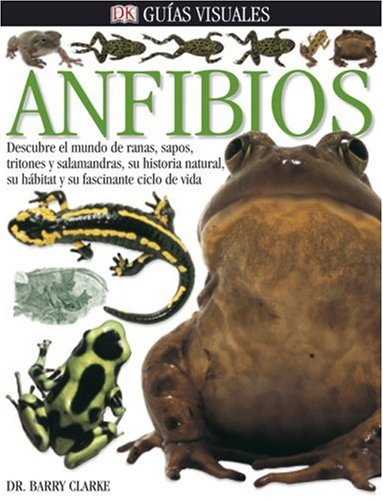The image is a detailed cover of a book on amphibians, featuring a predominantly white background with a horizontal black strip at the top. The black strip includes a reddish font "DK," set against an icon resembling an open book. Below this header, six various frogs are aligned horizontally. The green capitalized text "Amphibios" is prominently displayed beneath the frogs. Adjacent to this title, a large, close-up image of a green frog with black spots, appearing wet and slimy, occupies the right side of the cover. To the right of this frog, there's a black and yellow amphibian with distinctive markings on its body and limbs. Additionally, another frog, lighter green with black spots, is located below. There is a Spanish subtitle that reads, "Descubre el mundo de ranas, sapos, tritones y salamandras. Su historia natural, su habitat, y su fascinante ciclo de vida," describing the fascinating world of amphibians and their natural history, habitat, and life cycle. The bottom left corner features the author's name, "Dr. Barry Clark," in black letters.